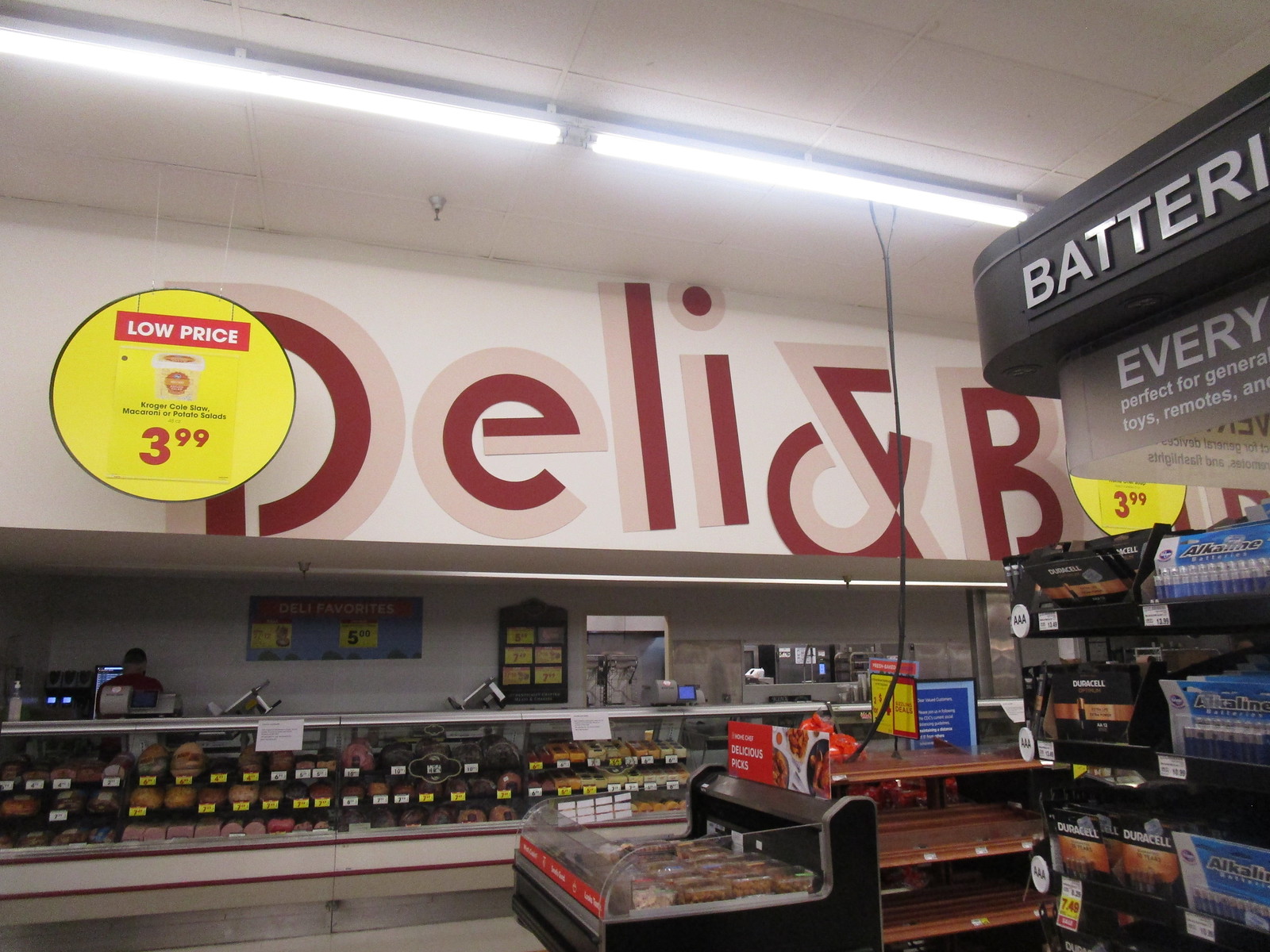The image is taken inside a grocery store, centered on a deli counter area. Dominating the middle foreground is a glass-fronted deli display case filled with an assortment of deli meats in varying shades of pinks, browns, and blacks on the left, and cheeses in different hues of yellow and white on the right, each with price tags. Behind the counter, a person, seen from the back, is wearing a baseball cap and a blue shirt, presumably a staff member attending to the deli section. Suspended from the white ceiling are bright white incandescent fluorescent light bulbs and a noticeable silver sprinkler head. Toward the back, a wall features a sign with red, stylized lettering that partially reads "Deli Ann" and a cut-off "B". Further to the right, mounted high, is a black rectangle with "battery" written in white, situated above a gray sign with partially visible white text reading "very". Adjacent to this are shelves presumably stocked with batteries. Prominently hanging from the ceiling on the left side is a circular yellow sign with "low price" in white letters, a partially recognizable product image, and "$3.99" at the bottom in red.